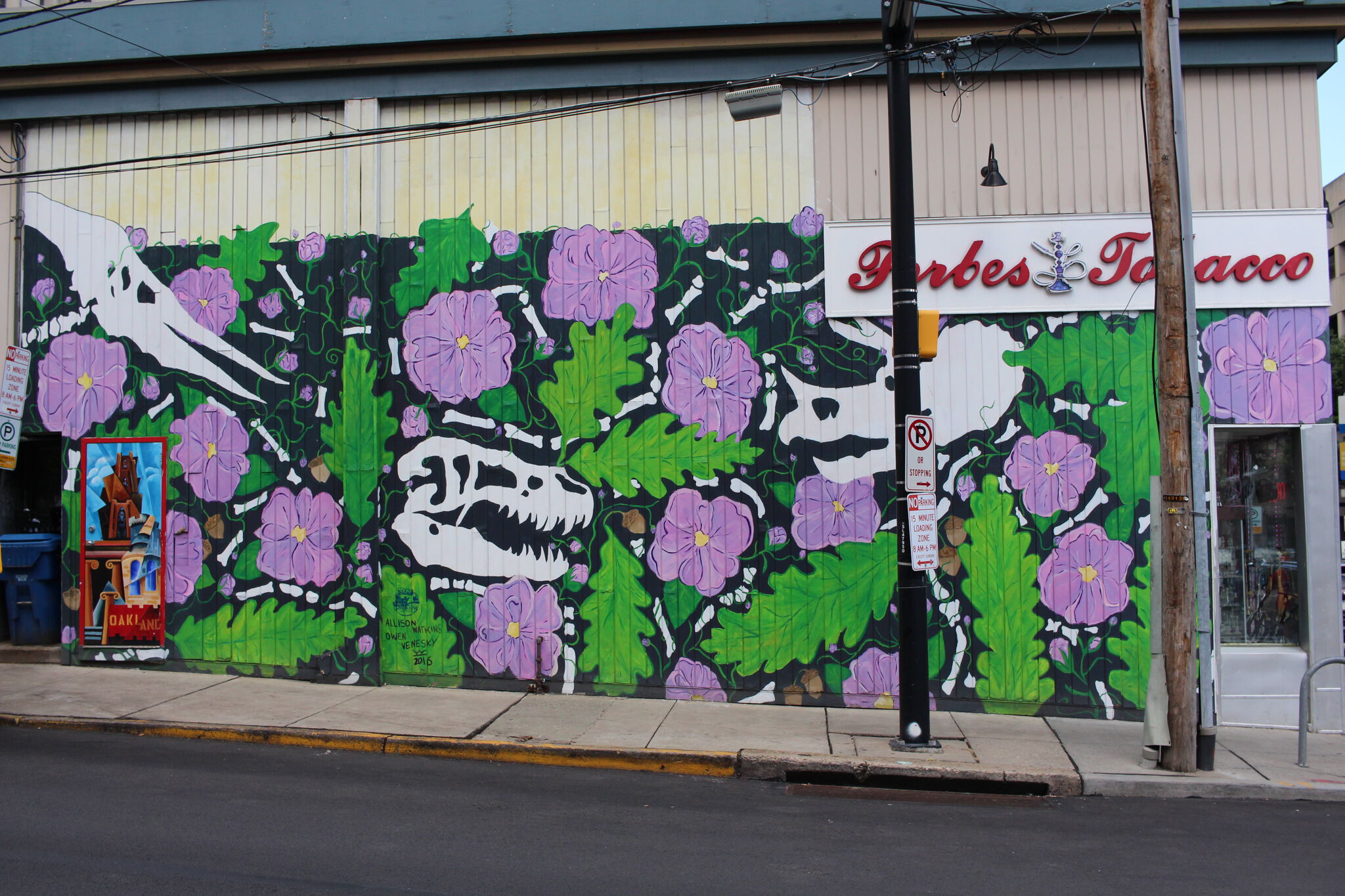The photograph captures a vibrant street corner scene, likely from an urban area. At the bottom of the image, there's a black, asphalt-paved city street. Adjacent to the street, a concrete sidewalk with large gray tiles extends alongside a low, single-story building, possibly a warehouse or store. The building is adorned with a colorful mural featuring an array of dinosaur skulls, blue and purple flowers, and green leaves, all set against a black background.

This mural covers the lower portion of the building, which also features yellow and light brown shutters. Above the mural, a banner reads "Forbes Tobacco" with an image of a hookah. A glass door is visible on the building's facade. The sidewalk is dotted with black and brown lampposts and electric poles, some bearing road signs such as "No Parking" and "No Stopping." A trash can is also positioned near the building, further detailing the urban environment.

The overall composition is enriched with the contrasting elements of the street, sidewalk, and the artistic mural, capturing a mix of functionality, urban grit, and creative expression.